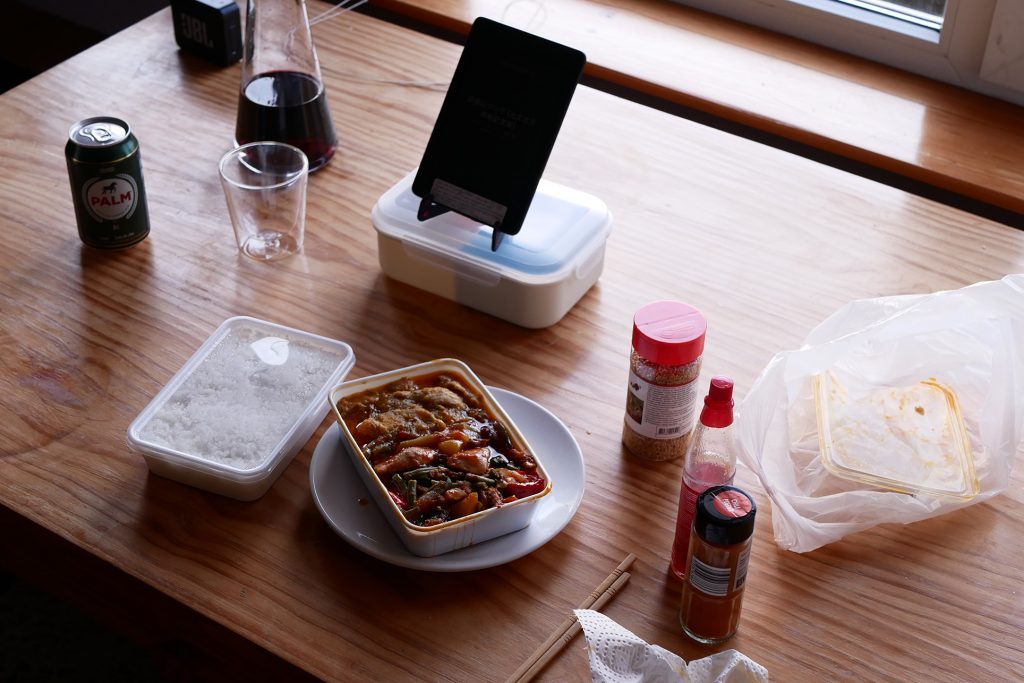In this image, a person stands in front of a wooden table, possibly at a restaurant, at home, or in a workplace break room. On the left side of the table, there is a glass beaker filled with a black liquid, likely soda. Positioned in front of the beaker is a large shot glass-like container, which appears to be made of either glass or plastic. To its left sits an unopened aluminum can featuring a white circle with red lettering that reads "Palm," accompanied by an image of a trotting horse, all set against a darker green background.

In the middle of the table, there's a plastic container equipped with a holder that looks suitable for propping up a phone to watch a movie. In the foreground, there is a clear plastic rectangular container holding white rice. Adjacent to it is a white ceramic or glass plate topped with a square arrangement of colorful vegetables—green and red—mixed with pieces of chicken and meat, all coated in a red sauce. To the right of the plate are a pair of wooden chopsticks.

Also on the right, there's a seasoning bottle with a red top, alongside another seasoning container that appears to be a small spray bottle. A white paper towel is positioned further to the right, and just off-camera at the top where the seasonings sit, part of a plastic bag can be seen, likely the bag that carried the food. Light shines through a window, indicating that the photo was taken during the day.